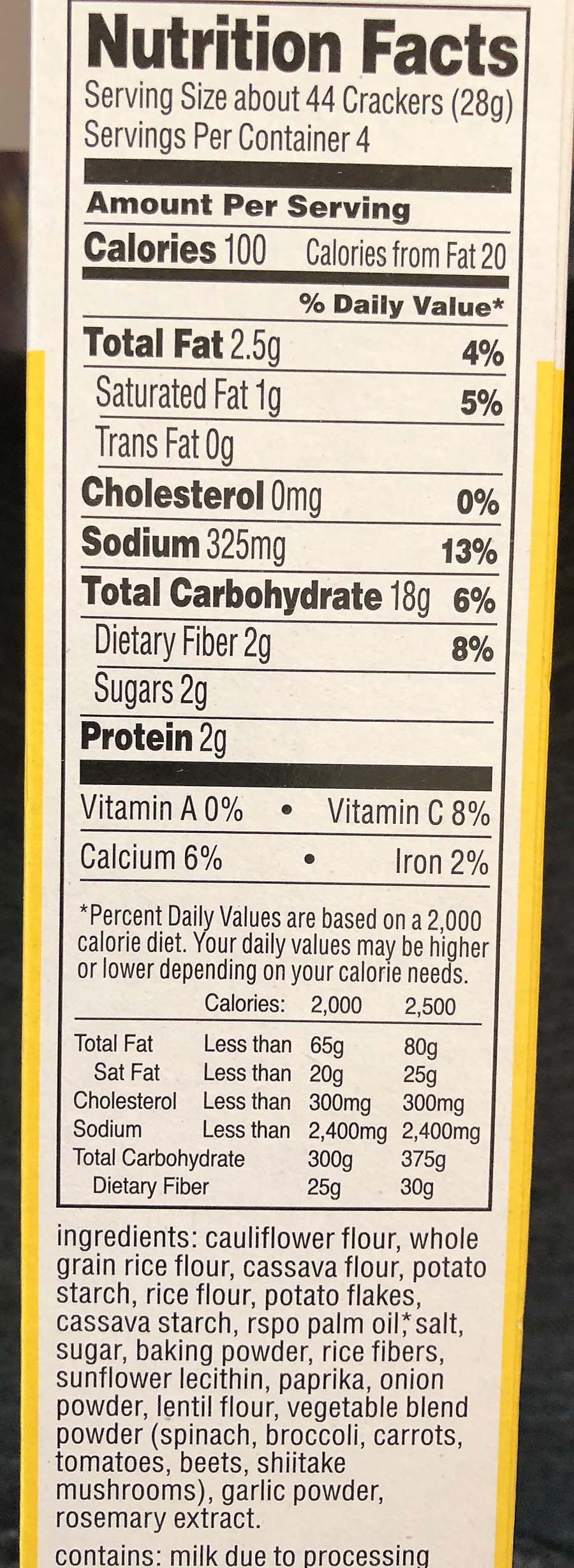This photograph features a detailed nutrition label on a box. The label, a long, slim rectangle, is displayed in an upright position. At the very top, bold black text reads "Nutrition Facts". Below, it specifies that the serving size is about 44 crackers (28 grams) and mentions that the container holds 4 servings. The label meticulously lists all the nutritional content in black text on a white background.

Under the header "Amount per serving," the label notes:
- Calories: 100
- Calories from fat: [Amount not specified]

Followed by detailed information on:
- Total fat
- Saturated fat
- Trans fat
- Cholesterol
- Sodium
- Total carbohydrate
- Dietary fiber
- Sugars
- Protein

Vitamin and mineral content includes:
- Vitamin A
- Vitamin C
- Calcium: 6%
- Iron

Beneath the nutritional values, the label provides a comprehensive list of ingredients, which includes: cauliflower flour, whole grain rice flour, various flours and starches, mushrooms, garlic powder, and rosemary extract.